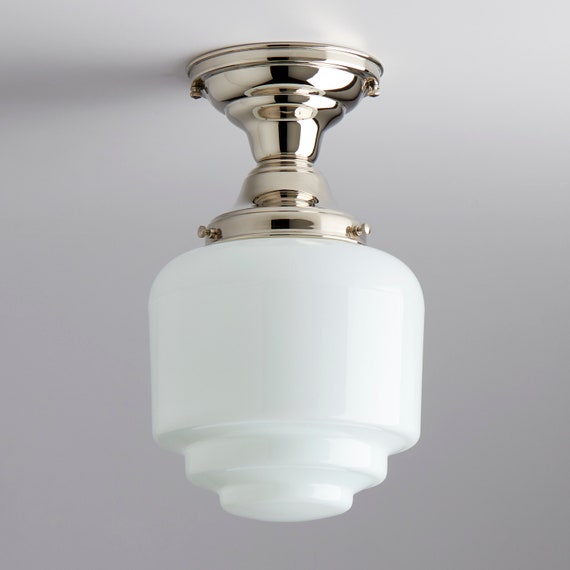The image showcases a small light fixture mounted on a solid gray ceiling. The fixture has a brass or gold-colored base, securely attached to the ceiling with visible screws. The base is reminiscent of a candle holder, featuring a design that widens at the top, narrows in the middle, and flares out again. Below the base, the light is covered by a decorative white glass piece that resembles the form of a rose without petals, characterized by a wider bottom that tapers upwards into a smaller knob and then flattens out. The white glass is opaque, not transparent, giving the fixture a delicate appearance that could shatter if struck. The entire setup presents a striking contrast against the plain gray background of the ceiling.